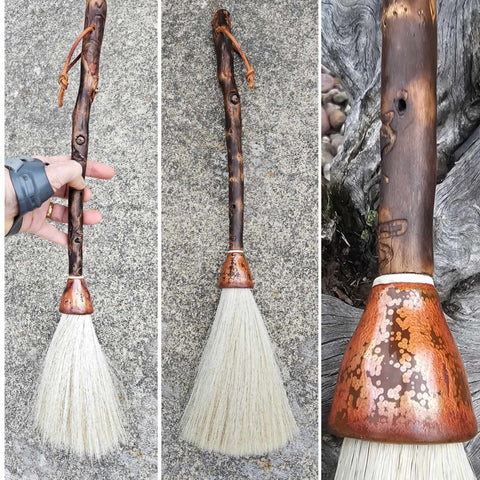This triptych features a series of high-detail photographs centered on a unique hand-crafted brush with white bristles. Each of the three equally-sized panels offers a different perspective on the brush, arranged against a neutral grey background, emphasizing its design and texture. The leftmost image presents a bandaged hand, wearing a wedding ring, grasping the wooden handle of the brush, showcasing a leather strap threaded through a hole in the handle. The middle image isolates the brush, leaning upright to highlight its full form and distinct white bristles. In the rightmost close-up, the focus is on the brush’s collar—the triangular section where the handle meets the bristles—revealing intricate details of its construction and the connection point, augmenting the tactile and visual craftsmanship of the object. The color palette across the photos includes natural tones of brown, black, grey, and white, subtly accented with a touch of gold, enhancing the brush's handmade aesthetic.